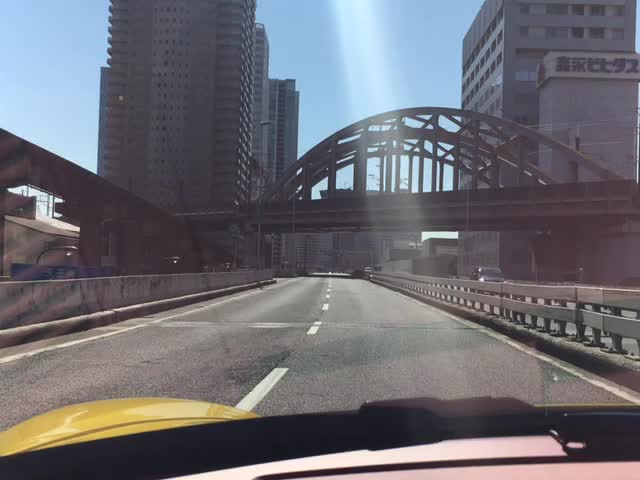A rectangular landscape image, slightly wider than tall, captures a view from inside a car driving down a two-lane road in an urban environment. This road, potentially an expressway in a city reminiscent of Pittsburgh, begins at the image's bottom edge and stretches upwards, gradually narrowing but never fully converging as it approaches the horizon. 

In the foreground, the dashboard and front end of the car are partially visible. The dashboard appears to be a mix of pink and black hues, while the left side of the hood is painted yellow, though the perspective makes it difficult to discern precisely.

The road itself is paved with light gray asphalt and divided by broken white lines. Both sides of the road are bordered by small railings. Beyond these railings, city buildings are visible, with two particularly tall commercial structures about 10-20 stories high standing prominently in the background on the left and right sides of the image.

Stretching across the center of the image from left to right is a small bridge, likely a footbridge, with two curved arches supported by poles. The bridge, constructed from dark metal, isn't imposing, standing about 15-20 feet high. Above it, the sky is light blue, adding a touch of tranquility to the urban scene.